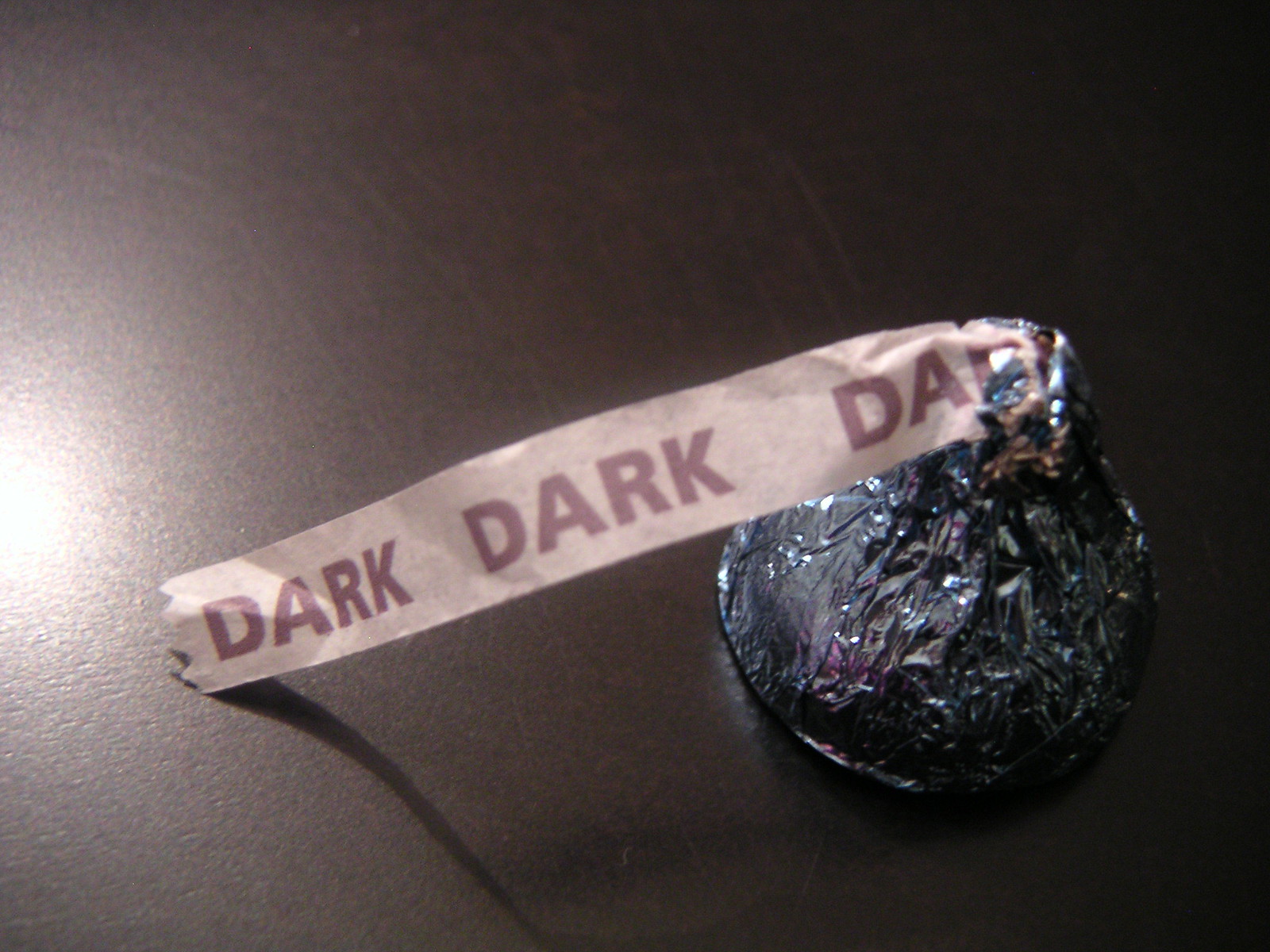The image depicts a dark chocolate Hershey's Kiss, wrapped in silver tinfoil, with a small beige paper tag protruding from the top that repeats the word "DARK" in dark brown letters. The Kiss is teardrop-shaped, also described as resembling a point on top, and is set on a dark brown countertop or table surface. The photograph appears to have been taken with a flash, as evidenced by the light reflections on the left side of the image, while the right side is predominantly in shadow. The light source is coming from above, creating reflections on the tinfoil, though the details of these reflections are indistinct.